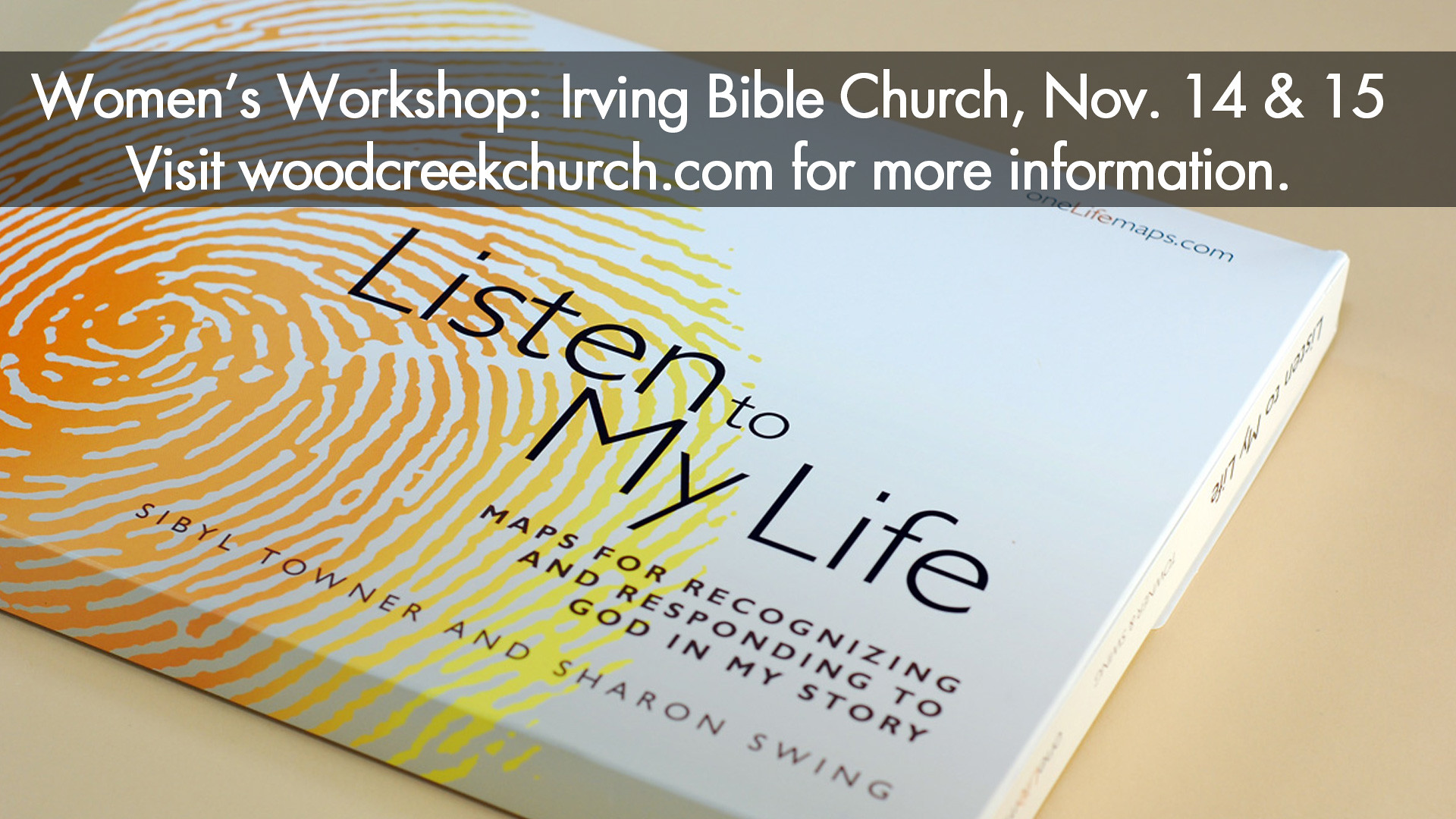The image resembles an advertisement or flyer for a women's workshop, set against a tan background. At the center is what appears to be a white box, perhaps resembling packaging, featuring an artistic fingerprint. This fingerprint displays a gradient that begins as a more intense orange and gradually fades to a lighter yellow towards the right side. The box bears a black text that reads, "Listen to My Life: Maps for Recognizing and Responding to God in My Story" by Sybil Towner and Sharon Swing. Towards the top of the image, a semi-transparent horizontal black bar spans the width, containing white text that announces, "Women's Workshop, Irving Bible Church, November 14 and 15. Visit woodcreekchurch.com for more information."